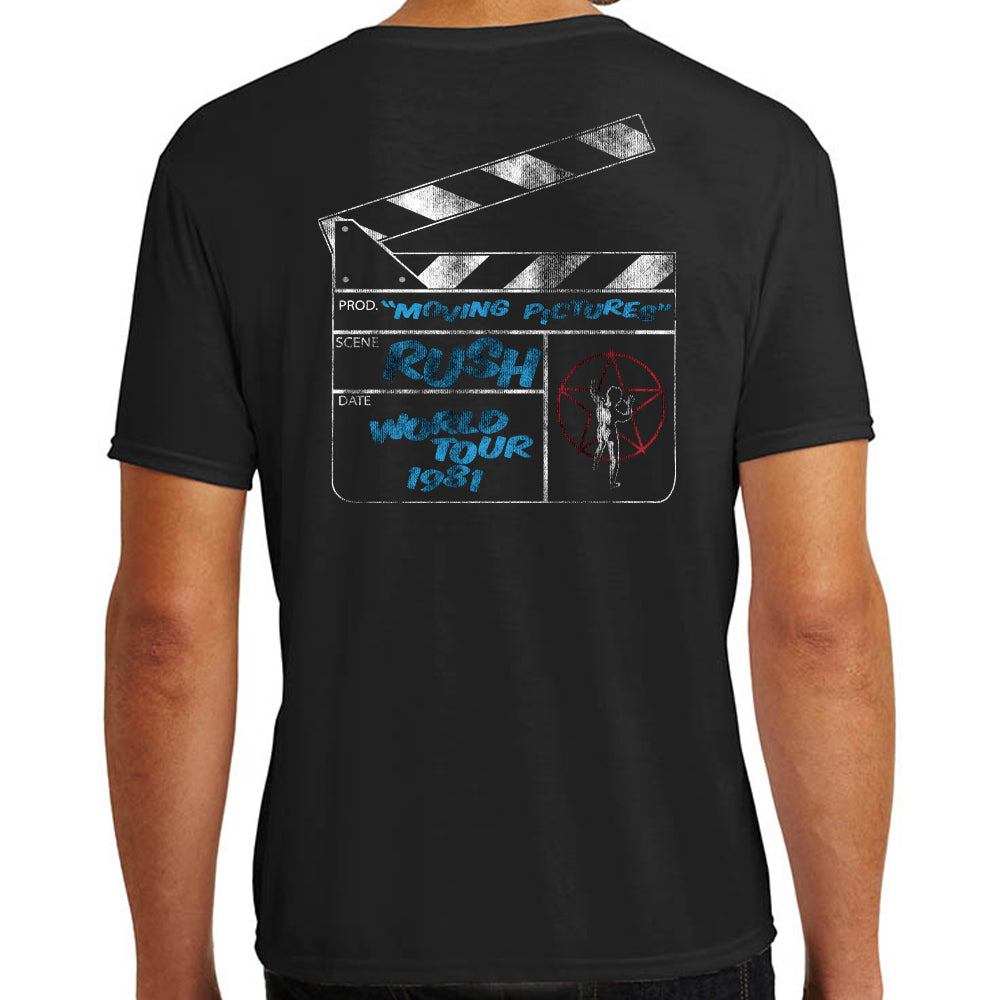This image is a digital photograph featuring a male Caucasian model wearing a short-sleeved, black cotton T-shirt. The background is a plain white, and the photograph appears to be about five to six inches high by four inches wide. The model is shown from the middle of his neck to about his hips, standing upright with his arms straight down to his sides. His light-tanned skin, with a slight reddish tone reminiscent of a mild sunburn, contrasts with the black T-shirt.

On the back of the T-shirt is an illustration of a movie director's clapperboard. The clapperboard consists of a central rectangle with a smaller, longer rectangle on top that features black and white diagonal stripes, resembling a ruler. Below the striped section is the text "P-R-O-D" in white. To the right, in large blue letters, it reads "Moving Pictures." The words "Scene," "Rush," (in blue uppercase text), and "Date" (all in white uppercase) precede the phrase "World Tour 1981" in blue text.

On the right side of the T-shirt's design, there is a red circle containing a blue pentagram and a black and white silhouette image of a man. The man's silhouette appears to be pushing against the star within the circle, adding an artistic element to the otherwise film-related graphics. Below this detailed image, the model is wearing dark blue or possibly black jeans.